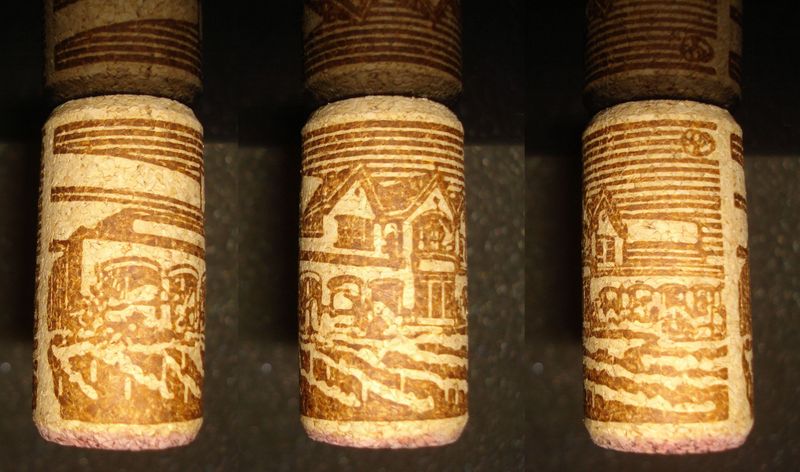The image is a zoomed-in view of three beige cylindrical objects that resemble corks, standing upright and attached to a wooden frame at the top. Each cork, about eight inches tall and four inches wide, features intricate brown drawings that depict various buildings and fields, possibly representing a winery. The objects have a textured surface that gives them a wood-like appearance. The leftmost cork shows a building with a pointy roof and a field in front, while the middle cork reveals more detailed aspects like doors and windows. Each drawing continues around the circumference of the cork, with some parts obscured due to the perspective. The overall composition suggests that the image may either reflect the corks in a mirror or show them through a side view.